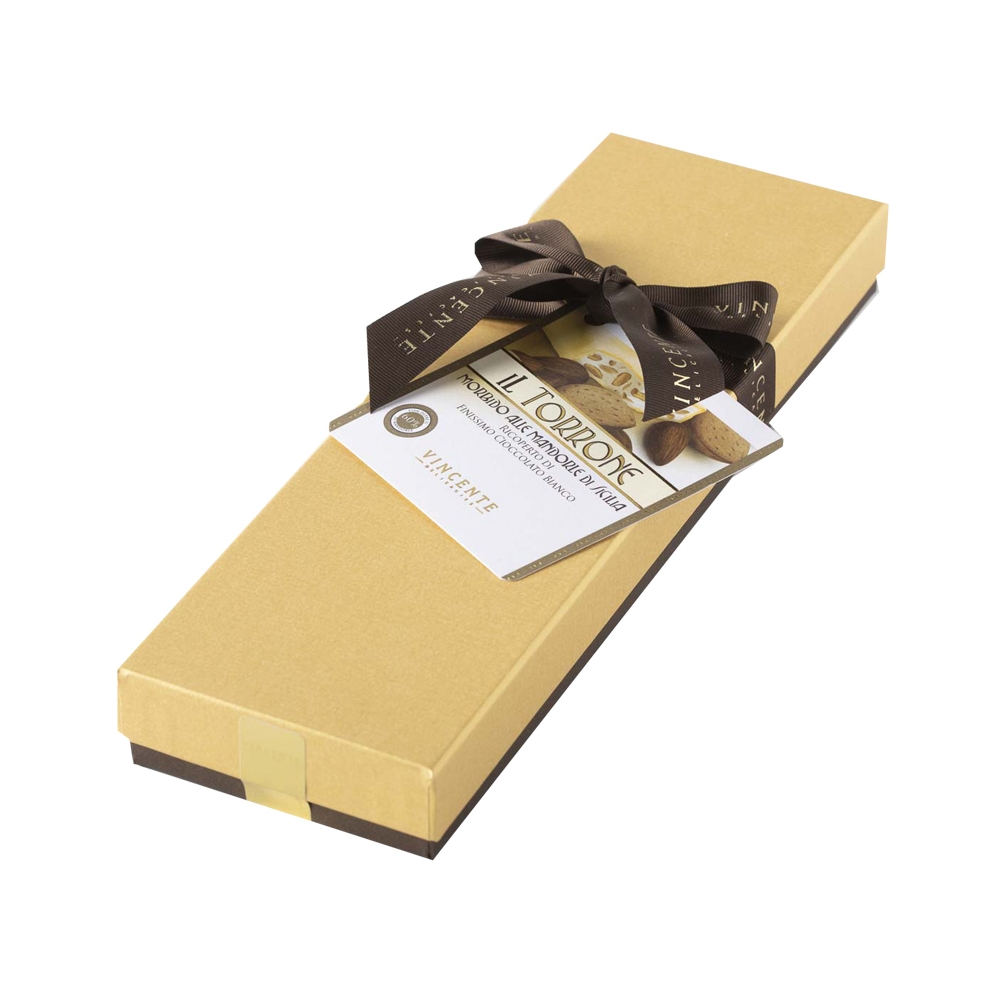This photograph features a sophisticated, long, rectangular gift box with a light brown and gold color scheme, set against a white background. The box is elegantly tied with a brown ribbon, which has "Vincente" printed on it, indicating the brand. A tag card attached to the ribbon reads "Il Torone," and further details in Italian - "morbido al mandorale di Sicilia" - suggest it contains fine Sicilian white chocolate with hazelnuts. The box also displays images of the chocolate and hazelnuts, reinforcing that it's a luxurious package of hazelnut-flavored white chocolates, handcrafted by Vincente, presumably in Italy.